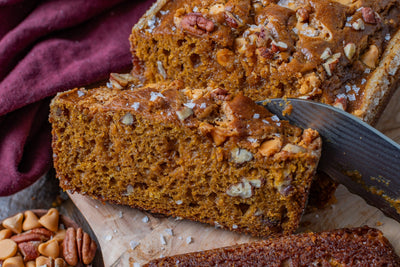The image is a small, horizontal rectangle photograph capturing a freshly sliced loaf of bread, most likely a pumpkin pecan loaf with peanut butter chips. The main loaf extends from the upper right, with its dark brown top sprinkled with nuts, possibly peanuts and pecans, and maybe a hint of sea salt. The loaf's sides are light brown, and its darker brown interior is filled with white and brown nuts. A sharp, silver knife, positioned from just below the middle on the right side, angles up and to the left, having just cut into the bread, leaving a slice to its left. The bread rests on white parchment paper. In the bottom right corner, an edge of another slice is visible. In the bottom left corner, there's a small bowl containing assorted nuts, likely including pecans and peanut butter chips. The upper left corner shows a piece of purple fabric, probably a hand towel, adding a splash of color to the scene. The entire setup suggests an indoor setting and a carefully composed arrangement on a wooden cutting board or serving platter.